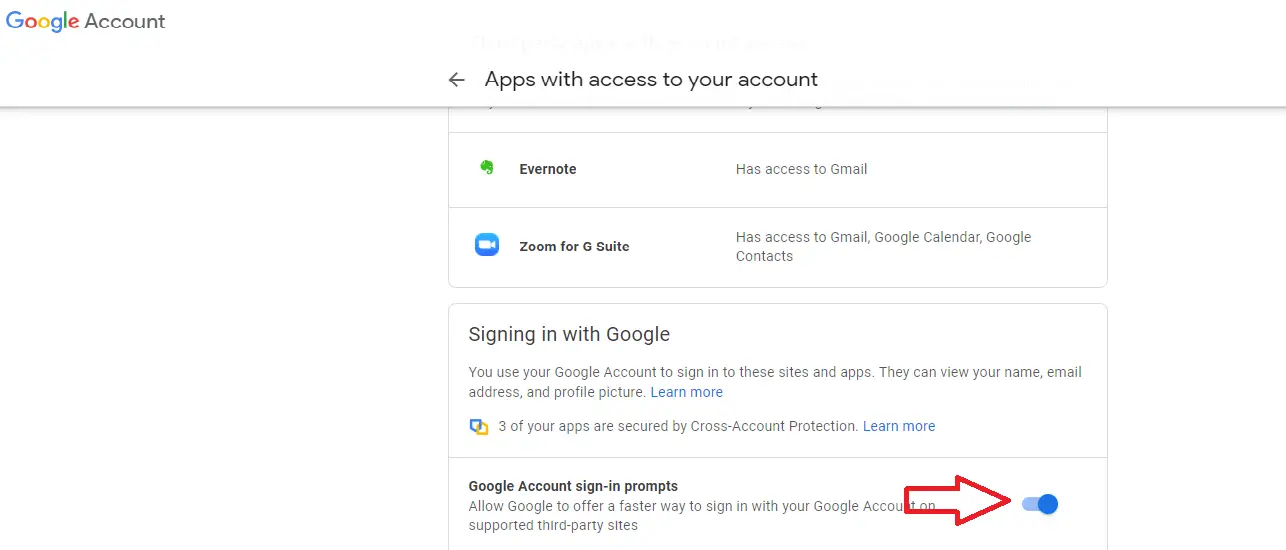This screenshot captures the "Apps with access to your account" section of a Google account settings page. The image showcases two distinct sections contained within separate boxes against a white background.

The first box lists applications that have access to the Google account. The partially included content reveals Evernote's entry, where the Evernote logo is displayed—a green elephant—and, to its right, the description indicates that Evernote has access to Gmail. Below this, a blue square icon with a white camera represents Zoom for G Suite, which has access to Gmail, Google Calendar, and Google Contacts.

The second box is titled "Signing in with Google" in bold text, with smaller text below it that explains, "You use your Google account to sign in to these sites and apps. They can view your name, email address, and profile picture. Learn more." Additionally, it mentions that "three of your apps are secured by cross-account protections. Learn more."

Another feature highlighted on the page is the "Google account sign-in prompts" option, which is toggled on, signified by a blue switch and emphasized by a red arrow pointing directly at the toggle button.